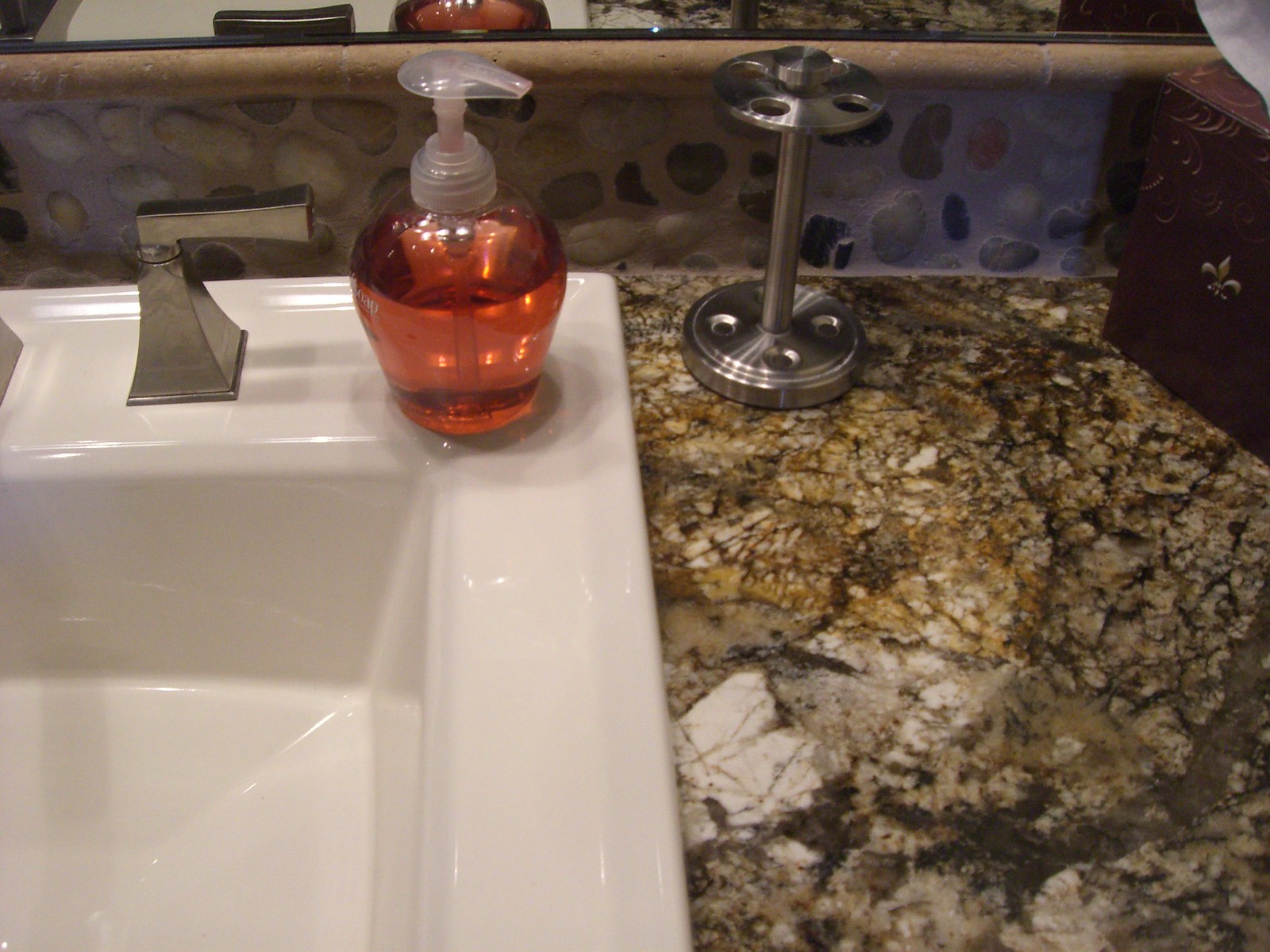This image showcases a modern, integrated washbasin in a bathroom, seamlessly moulded as part of a single sink top. The material appears to be ceramic or plastic, enhancing its sleek and unified appearance. Positioned centrally on the washbasin is a unique tap that evokes the nostalgic design of a miniature gramophone horn, lying on its side. To the right, there is a large glass jar filled with an orange liquid, equipped with a pump top, presumably for soap or hand lotion.

The floor below presents an unusual and eye-catching design, featuring a chaotic mix of yellow and white patterns, creating a whimsical and somewhat perplexing visual effect. Adjacent to the washbasin, a chromium-plated stand catches the eye with its industrial aesthetic. This stand features a base and a circular top, both punctuated with multiple holes, though its precise function remains unclear due to the absence of items in the holes.

On the right side of the scene, a brown cupboard stands with its door slightly ajar, revealing a metal fleur-de-lis symbol on its surface, adding an unexpected touch of elegance and mystery to the overall setting.